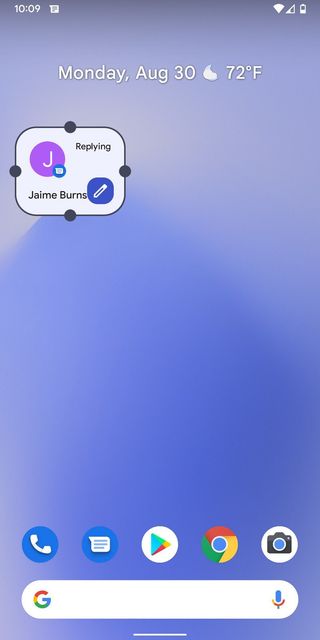The image captures a detailed view of a smartphone screen with a predominantly blue background intertwined with subtle gray hues, creating a smooth, visually pleasing gradient. 

In the top left corner, the digital clock displays "10:09". On the top right, there are essential status icons: a wireless signal indicator, cellular signal bars, and a battery icon showing less than half charge.

Beneath this, in crisp white text, it reads "Monday, August 30." Just below, there is a weather widget displaying an icon resembling a cloud with a temperature of "72°F."

Further down on the left side of the screen, a small rectangle with a black border and black dots in the middle of each side encloses some more details. Inside the rectangle, there is a circle with a purple background featuring the white letter "J," next to which the word "replying" is written. Below this, the name "Jamie Burns" is displayed. To the right of this name within the same rectangle, against a blue background, a pencil icon is present. 

At the very bottom of the screen, five primary icons are horizontally aligned: a phone icon, text messaging icon, Google Play Store icon, Google Chrome icon, and a camera icon. 

Below these icons, the Google search bar is centrally placed with the recognizable "G" logo on the left end, and a microphone icon on the far right end of the search bar, indicating voice search functionality.